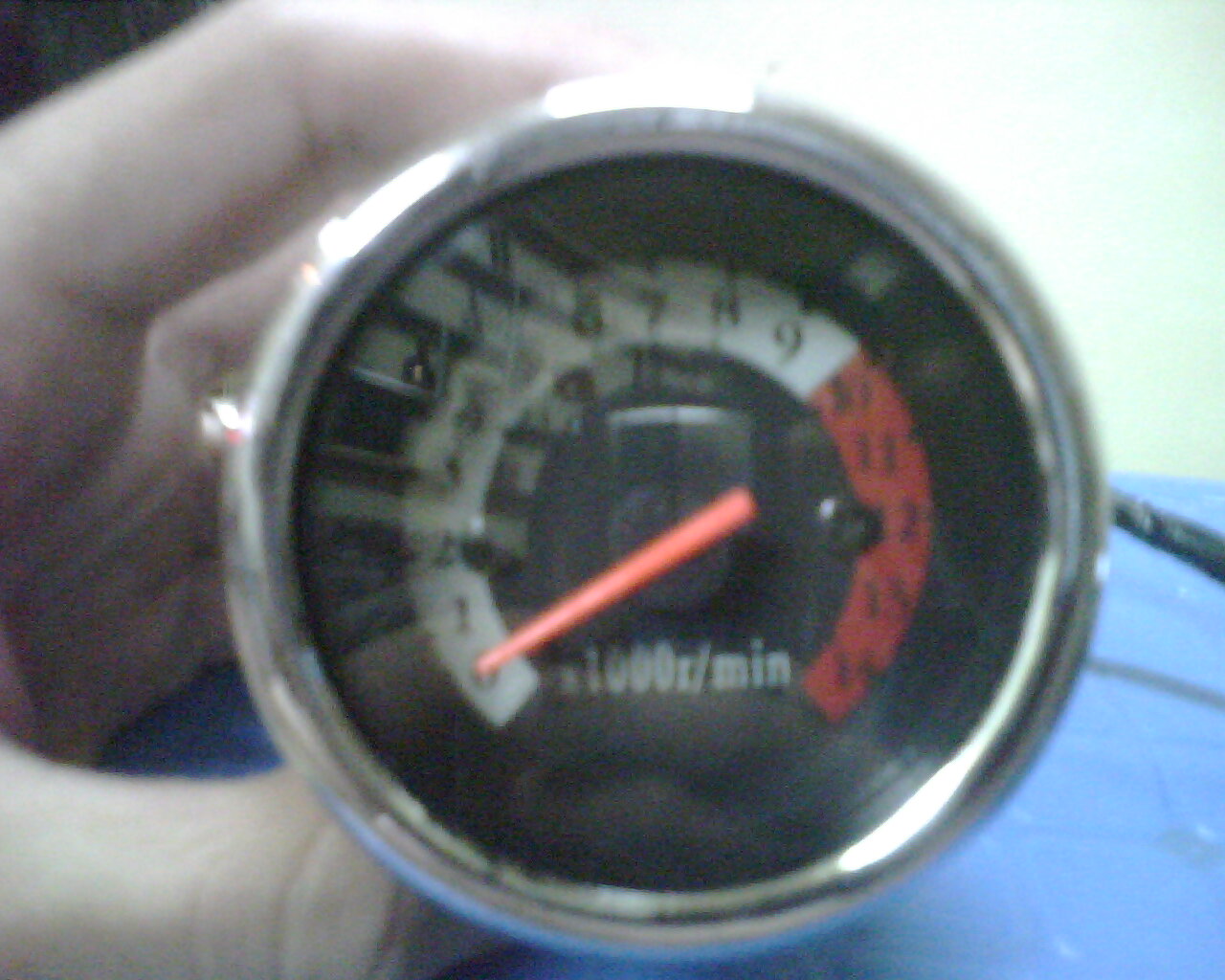The image depicts a close-up of a round, metal measurement gauge, held by a hand that rests on a blue surface. The gauge features a black face with numbers inscribed around its circumference, ranging from 0 to 9 on a white background, while the remaining numbers appear on a red background. The red needle, positioned prominently on the gauge, indicates a specific measurement. Just below the needle, there is text inscribed in the gauge that reads "1000 R per minute." The image quality is slightly grainy and blurry, which obscures some of the finer details on the gauge.